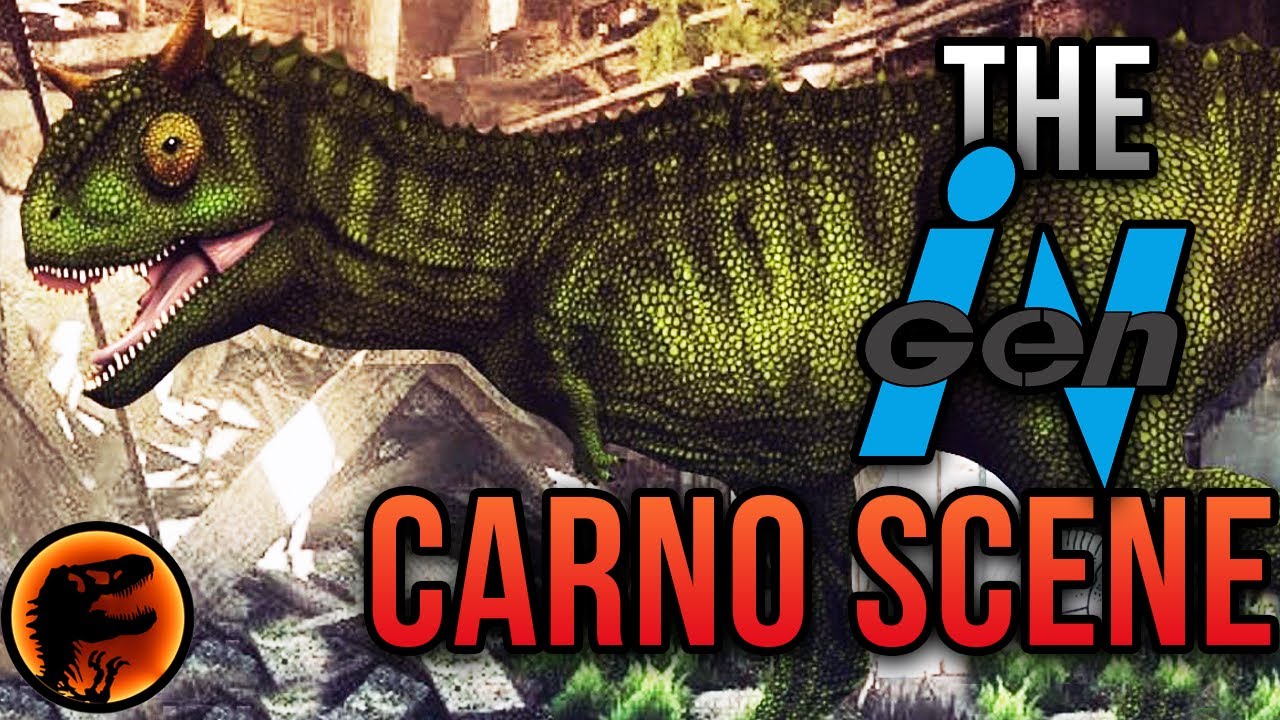This advertisement image, measuring approximately 5 inches wide by 3 inches high, predominantly features a green-scaled dinosaur with various striking attributes. Positioned from the upper left across to the right and taking up about half the top of the image, the dinosaur flaunts short front arms, a pair of brown horns on either side of its head, and a fearsome open mouth revealing numerous short white teeth and a long pink tongue. The dinosaur’s yellow, gecko-like eye and black stripes running down its back add to its vivid depiction.

On the right side of the image, text extends from the top right to the bottom. The text reads "The InGenCarno scene," with "Carno scene" presented in bold red capital letters. The word "the" is in bold gray print with a black outline, followed by "InGen" in smaller gray text across blue and the red "Carno seen" also featuring a black outline. 

In the lower left-hand section of the image, there's a distinct circle. Within this circle, set against a reddish-orange background, is a black silhouette of a dinosaur, likely a T-rex, with its mouth open and front hands visible, creating a striking contrast to the vibrant surrounding elements.